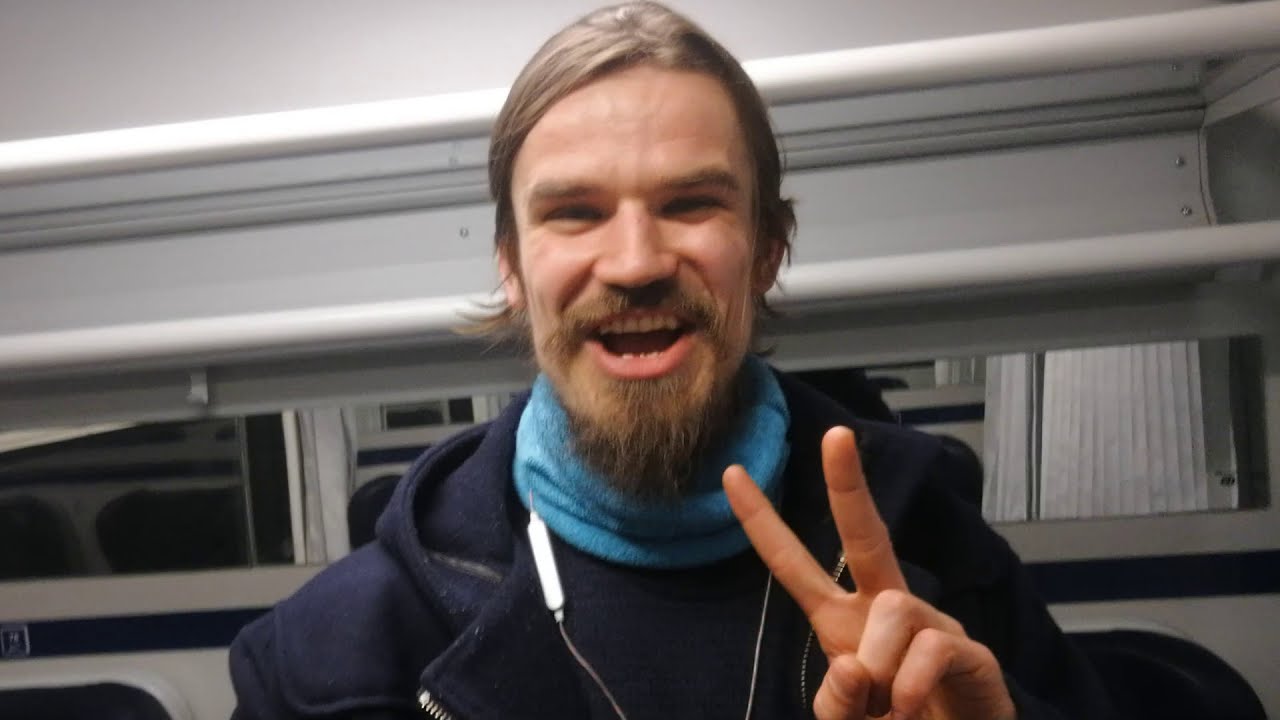This image depicts a joyous man with a neatly groomed brown beard and long hair pulled back, possibly into a ponytail. He is front and center in the frame, donned in a dark navy blue hooded sweatshirt and a light sky blue scarf wrapped around his neck. A pair of white earbuds is visible, either tucked into the scarf or hanging freely around his neck. The man displays a wide, enthusiastic smile, his eyes partially closed from the joy he's expressing, and he’s holding up a peace sign with his left hand.

The background suggests a setting inside a train, indicated by the presence of an overhead storage compartment behind him, possibly for luggage. There is also a curtain visible, which might partition a private area or a sleeping car, further hinting at a travel context. A light source shines from behind his head, adding a gentle glow to the scene. There are no textual elements in the image, allowing the vivid colors and the man's exuberant expression to take center stage.